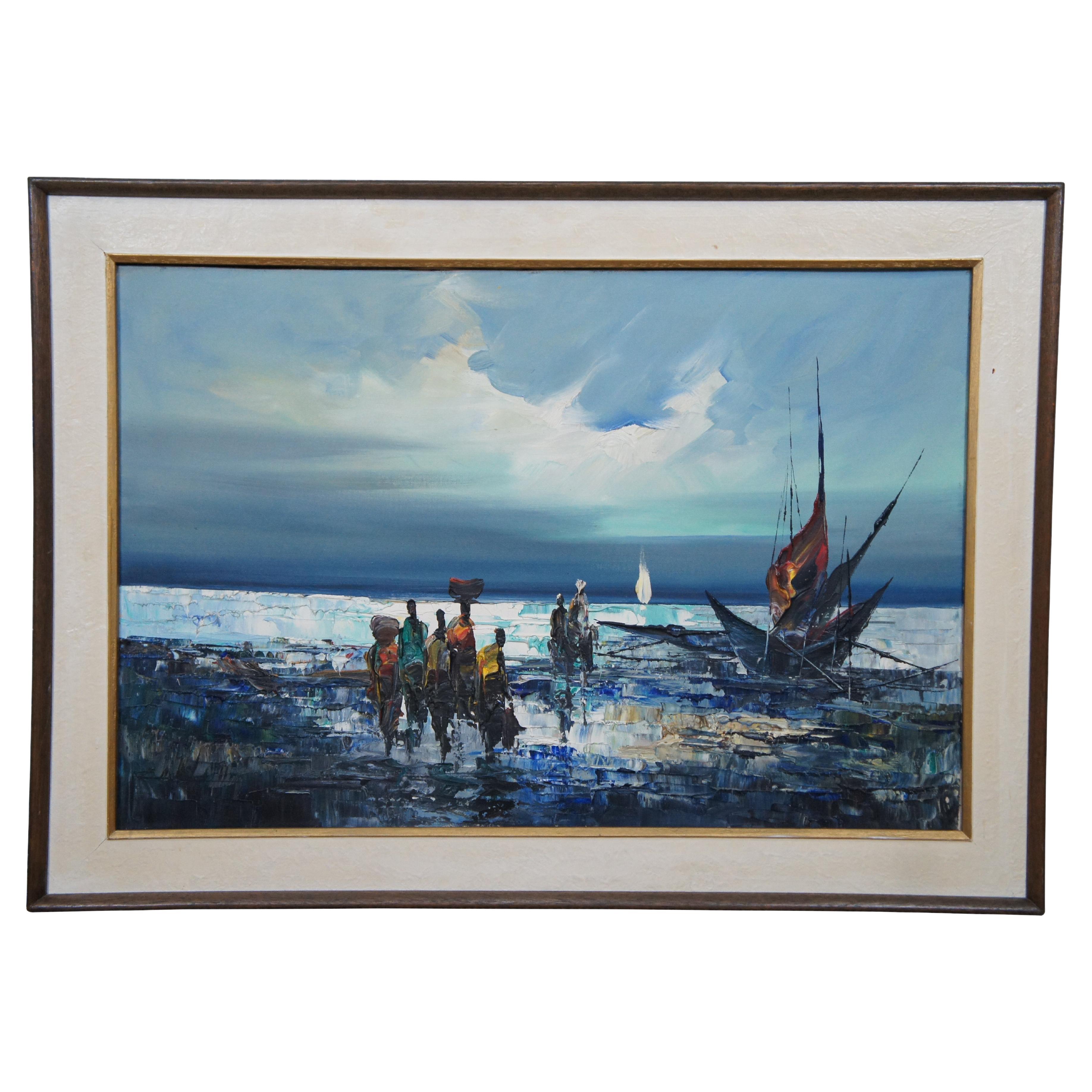The painting artistically captures an African scene in an impressionistic style, featuring a ship that has either come ashore or wrecked in the water. This ship, with its distinct angular design and orange sail, is situated against a backdrop of a dimming blue evening sky, where the sun is just starting to break through the clouds. In the distance, another white-sailed ship can be seen. 

In the foreground, five dark-skinned figures move towards us, their forms accentuated by colorful scarves and soft muted hues of yellow, orange, and blue. These figures, possibly representing a family, immigrants, or fishermen, are depicted carrying baskets on their heads while wading through the water. The painter has utilized a color palette of dark blue, light blue, gray, and beige, creating an ocean-like scenery with dark brush strokes in the foreground. The overall scene is framed by a brown and golden-brown border, adding a touch of elegance to this evocative piece.